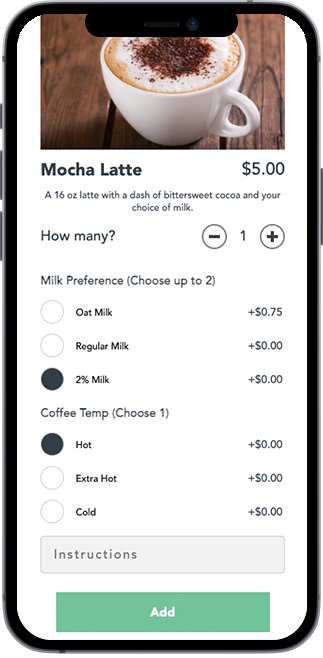A detailed and descriptive caption for the image could be:

---

A high-quality photograph captures a smartphone displaying a mobile app or website with a sleek, minimalist design. The phone screen shows a shopping interface featuring a drink selection. Against a light white background, prominently at the top, is an enticing image of a mocha latte in a white ceramic cup placed on a table. The latte features a rich foam dusted with what appears to be bittersweet cocoa powder, giving it a dark brownish-red hue.

Below the eye-catching picture, the text reads "Mocha Latte - $5.00" and provides a mouth-watering description: "A 16-ounce latte with a dash of bittersweet cocoa and your choice of milk." 

Further down, the interface offers the option to select the quantity, currently set to one, with clickable plus and minus buttons for adjustment. Following this, users can specify their milk preference, with choices including oat milk, regular milk, or 2% milk, of which 2% milk is selected. 

Additionally, there's an option for determining the coffee temperature, choices being hot, extra hot, or cold, with the current selection being hot. 

Beneath these options, there's a text box inviting users to add any special instructions for their order. The interface is designed for a seamless user experience, ending with a prominent green button labeled "Add to Cart," ready for the user to complete their selection.

---